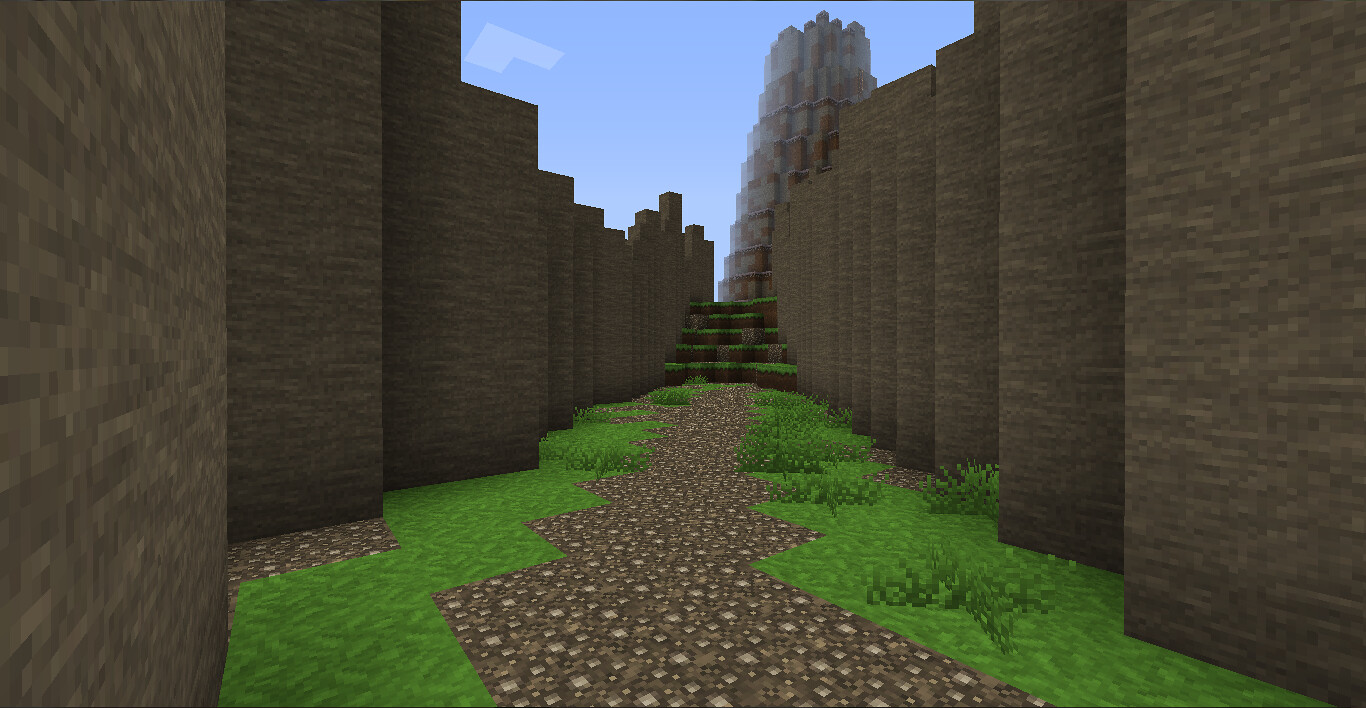The image appears to be a scene from the video game Minecraft, characterized by its pixelated, blocky style. The scene features a courtyard with green, digital grass flanked by high brown brick walls on both sides. These walls are set at an angle and create a corridor effect. In the center of the courtyard, a zigzagging cobblestone path lined with clumps of grass and bushes leads to a set of stone steps. Each step is also covered in grass, adding to the lush, green appearance. The stairs ascend towards a large, cylindrical tower made of brown and gray blocks, standing tall and prominent in the background. Above this tower, the sky is light blue, adorned by a single L-shaped white cloud.